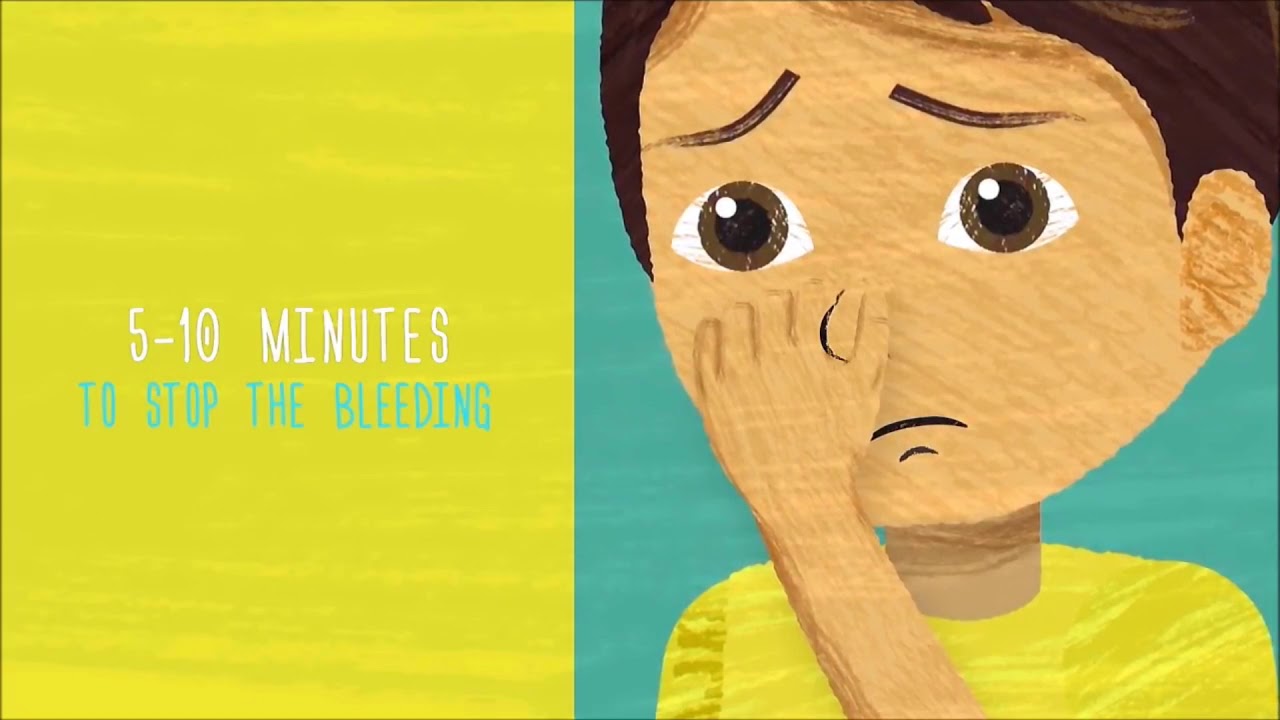The image is a detailed illustration divided into two sections. On the left, a vertical yellow rectangle bears the text "5 to 10 minutes to stop the bleeding," with "5 to 10 minutes" in white and "to stop the bleeding" in blue or green. The right side features a cartoony painting of a sad-looking boy with brown hair, brown eyes, downturned eyebrows, and a simple line for a mouth, suggesting sadness. He has light skin and distinctly rounded ears and facial features. The boy is holding his nose with his left hand, presumably to stop a nosebleed. He wears a yellow shirt, and his background is a light blue or turquoise color. The overall style resembles a marker or watercolor rendering typical of children's illustrations, aimed at teaching kids how to handle nosebleeds without panicking.